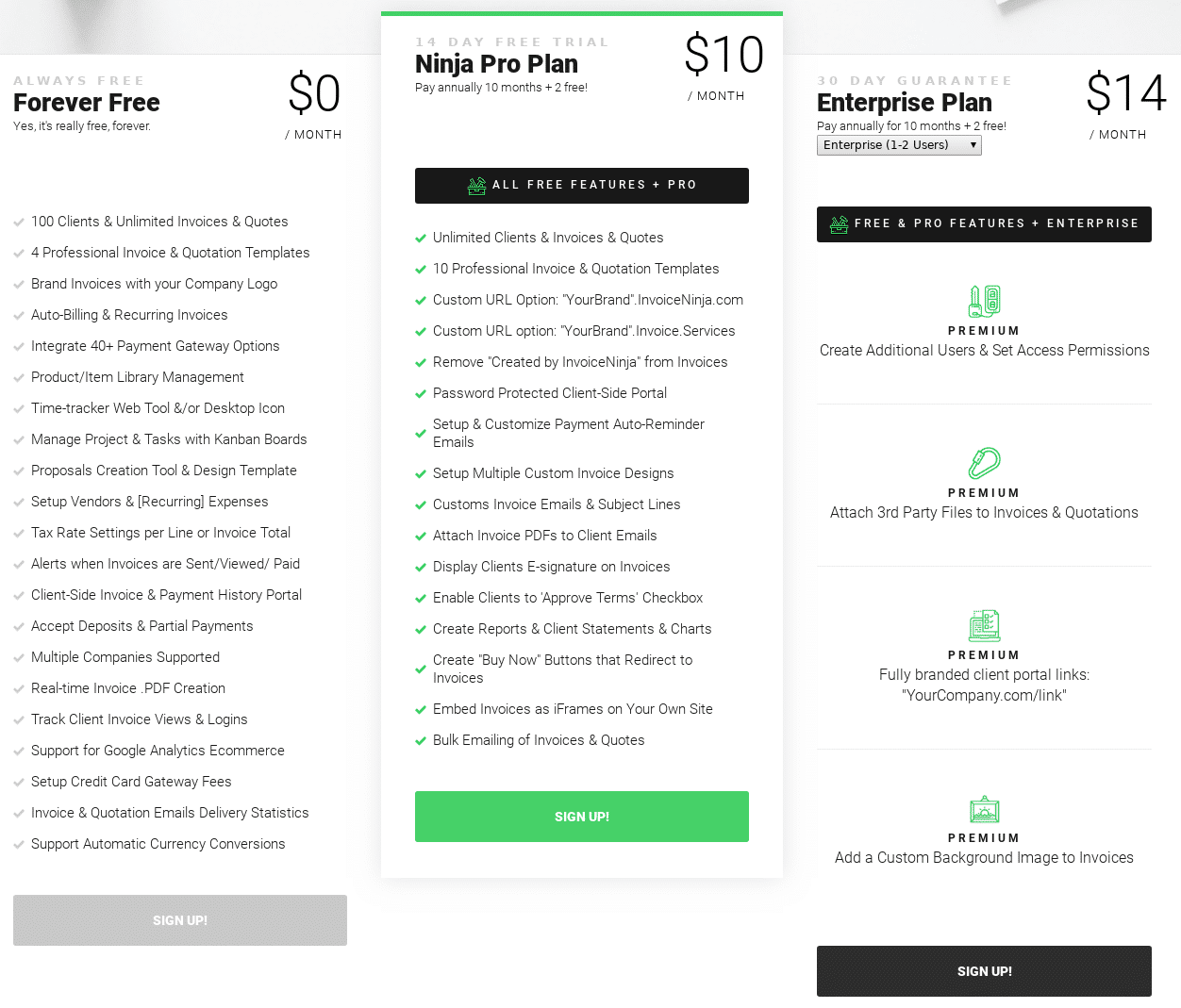This image, set against a solid white background, features three separate screenshots presented side by side. The leftmost screenshot showcases a pricing plan titled "Forever Free" written in bold black text. At the upper right of this section, "Zero dollars a month" is noted. Below, a list of features is presented, each marked with a gray check mark. The features include "100 clients," "Unlimited invoices and quotes," "Professional invoice and quotation templates," "Brand invoices with your company logo," and "Product item library management." Beneath this list is a gray action button with the text "Sign Up" displayed in white.

The middle screenshot features the "Ninja Pro Plan" heading in bold black text. In the upper right corner, the cost is noted as "Ten dollars a month." Below this, a black banner with white text states, "All free features pro."

The rightmost screenshot pertains to the "Enterprise Plan," displayed in bold black text. The upper right corner highlights the cost as "Fourteen dollars a month." The layout and design elements mirror those of the previous plans, providing a cohesive comparison between the different pricing tiers.